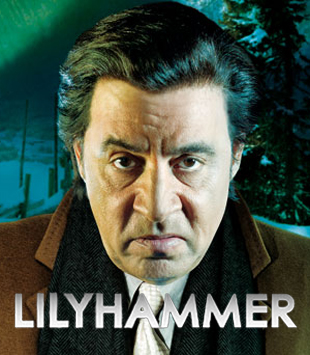This photograph features a man with dark, wavy hair brushed back, revealing his entire forehead. His expression is stern as he gazes directly at the camera, with deeply furrowed eyebrows and two pronounced wrinkles between them. The dramatic lighting highlights the intricate lines on his forehead and face, emphasizing his intense frown. He is dressed in a large, brown coat over a black scarf, complemented by a white button-up shirt and a grey tie, reminiscent of a gangster's attire. In the background, there is a snow-covered tree, and the scene is enveloped in a dark, greenish hue, enhancing the moody atmosphere. The word "Lilyhammer" is printed across his chest area. His brown eyes and the bags beneath them are accentuated by side lighting, which casts dark shadows across his face, adding to the overall dramatic effect.